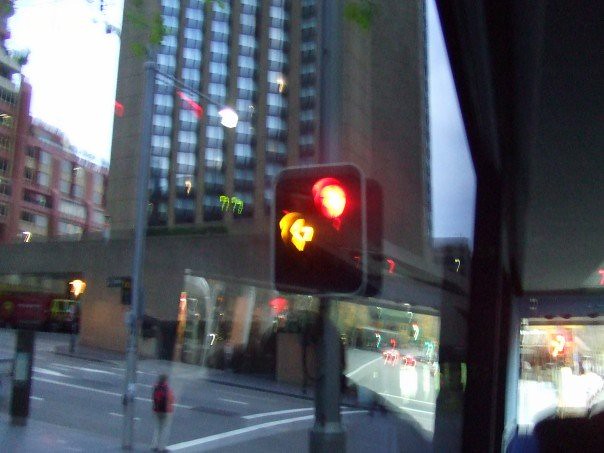The image appears to be taken from the window of a double-decker city bus, looking out onto a bustling urban street. The picture is slightly blurry, likely due to the reflection and movement of the bus. Prominently featured in the center of the shot is a high-rise brick building with numerous dark windows, flanked by other distant structures under a light blue sky with hints of white clouds. A person dressed in a black top and khaki pants stands at the street corner, ready to cross the road. Visible street markings and traffic lights enhance the urban scene; the traffic light displays a red signal alongside a yellow left turn arrow. Reflections in the bus window create distorted, reddish-orange shapes that resemble the number seven, adding a surreal, subdued quality to the photo. The edge of the bus window and someone’s dark brown hair can be seen in the lower parts of the image, capturing a slice of everyday city life.